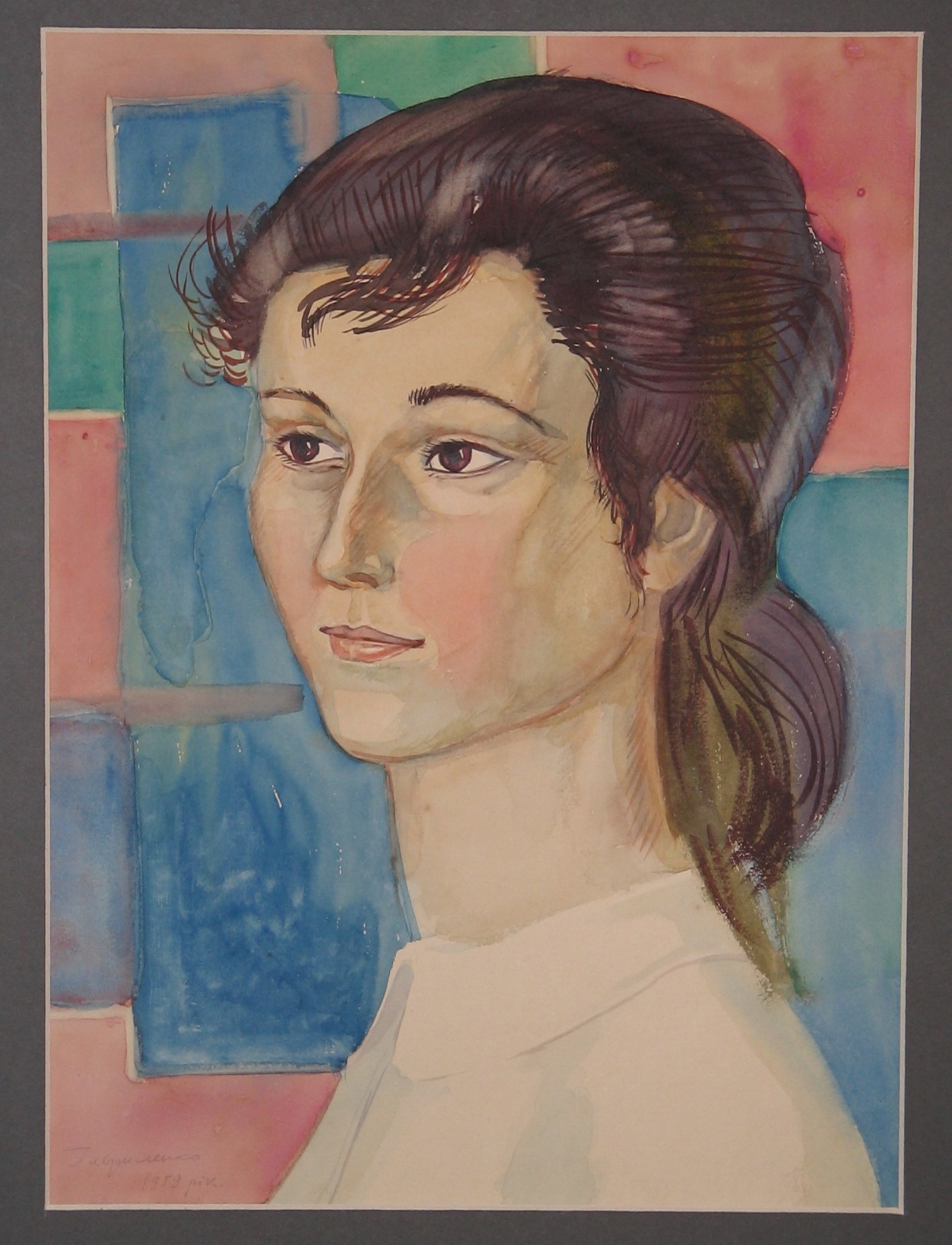The painting depicts a profile view of a woman angled slightly towards the painter. Her chestnut brown hair, which is relatively pulled back with a few wispy bangs, cascades longer at the base of her neck. She features brown eyes, thin eyebrows, a sharp European nose, and small, thin pink lips. Her neck is exceptionally long, and she wears a cream-colored, high-collared shirt that creeps up her neck.

The background appears abstract, consisting of a patchwork collage of washed-out colors, including red, blue, and green rectangles, with notable squares of blue that may suggest a sky or light filtering through a frosted or coated window. The colors and shapes behind her provide an unrecognizable, visually abstract backdrop, adding an intriguing, almost ethereal quality to the composition. The woman's head tilts slightly to the left, while her eyes gaze towards the right, capturing a moment of introspective thought in this detailed and textured portrait.